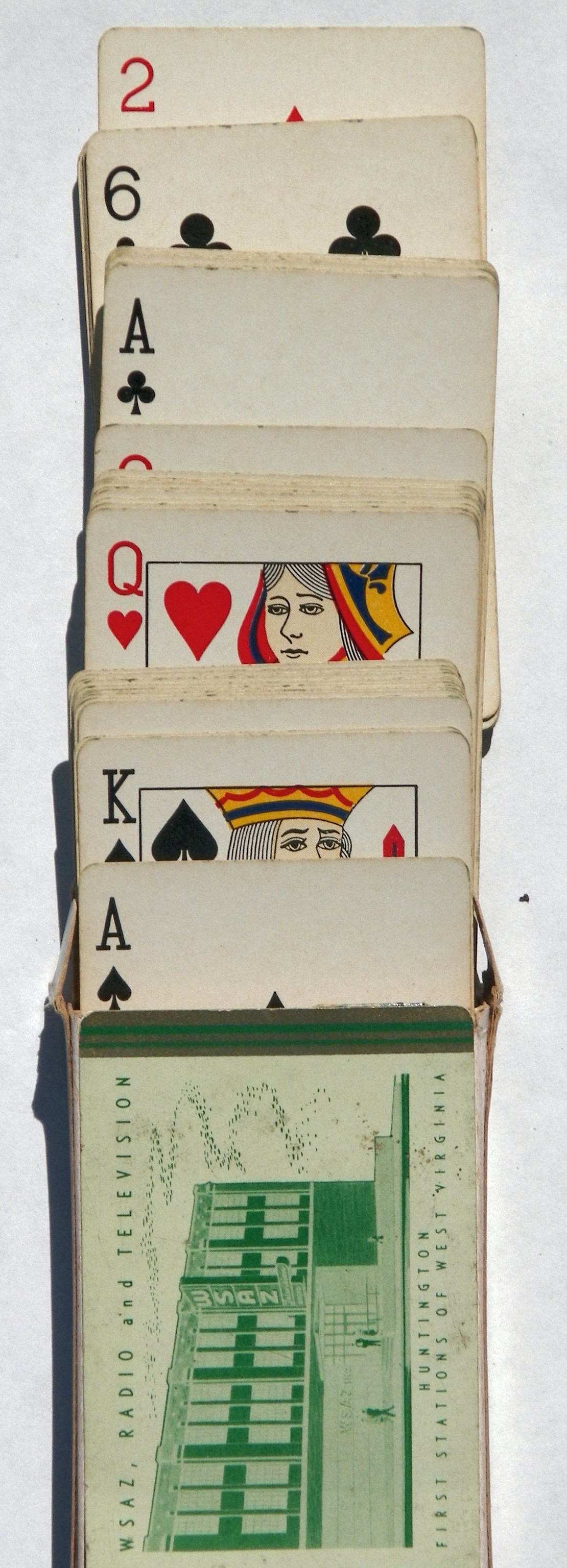This photograph captures a top-down view of an opened deck of playing cards, with the cards pulled out vertically and unevenly spread. The cards appear in staggered layers, revealing individual ranks and suits at various heights. At the top, a few cards are prominently visible, starting with the two of diamonds. Just below, the six of clubs is discernible. Further descending into the stack, the ace of clubs is slightly revealed.

In the layered arrangement, a single card with a hint of red peeks out inconspicuously, adding a touch of mystery. Another small stack of cards exposes the queen of hearts on its surface. Below this, another stack shows a glimpse of the king of spades. Descending further, the ace of spades is partially exposed, with only the top quarter visible against the cascade of cards.

The deck’s box, a thin cardboard container, lies at the base. It features a light green color with darker green artwork depicting the side of a building. The building's sign reads "WSAZ," and additional text on the box states "WSAZ Radio and Television" at the top and "Huntington First Stations of West Virginia" at the bottom. The background of the photograph is a blend of white and light gray tones, which subtly complements and highlights the detailed card arrangement.